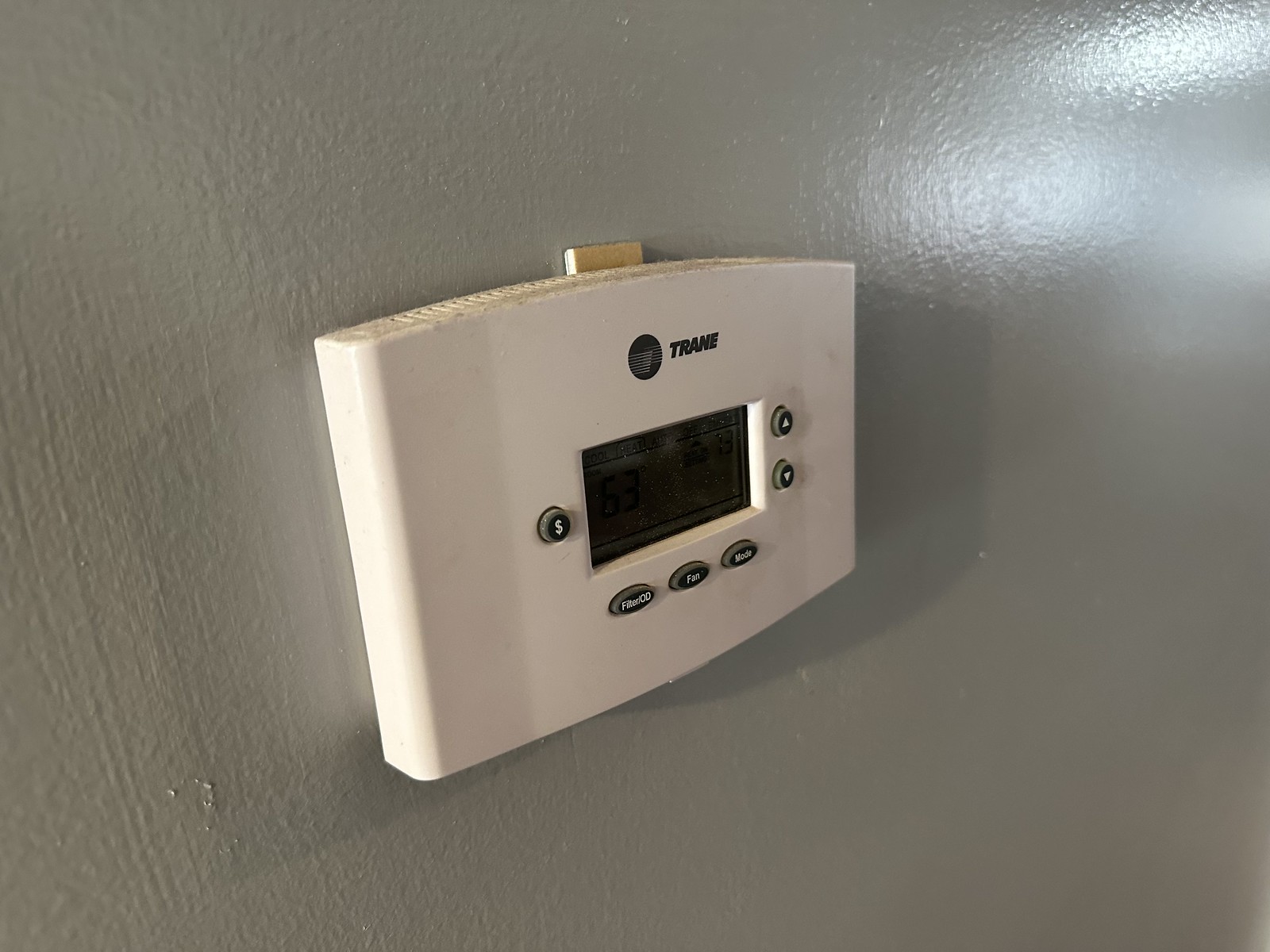A close-up photograph of a thermostat attached to a grayish wall. The thermostat is a rectangular shape with subtly curved edges at the top and bottom, giving it a dimensional appearance. The device is predominantly creamy white, featuring a small, unlit black digital screen in the center. The brand name "Trane" is prominently displayed below a circular, black emblem at the top. On the left side of the screen, there is a button marked with a capital "S." To the right of the screen, two buttons are positioned vertically: an up arrow and a down arrow. Additionally, at the bottom of the thermostat, there are three black oblong buttons with white text, though the inscriptions are not legible. A layer of dust is noticeable at the top, suggesting that the thermostat has not been cleaned in some time.